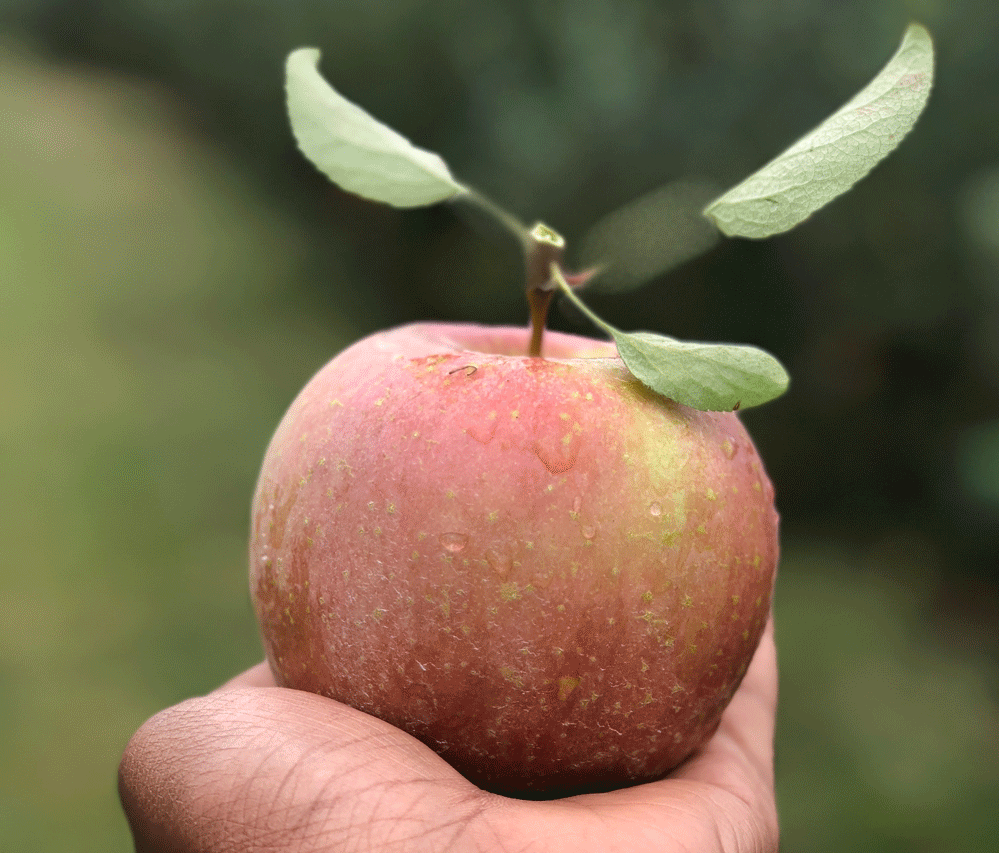This photograph captures a close-up view of a freshly picked apple resting in a medium-dark toned hand that is facing away from the camera. The apple, which exhibits a pinkish-red color with hints of green and yellow hues, appears freshly washed with water droplets glistening on its surface. A brown stem emerges from the top of the apple, accompanied by three to four green leaves, enhancing its natural appearance. The background is a soft, out-of-focus blur, featuring green hues that suggest a natural landscape with grass, trees, or possibly an apple tree, adding to the fresh, just-harvested ambiance of the image.